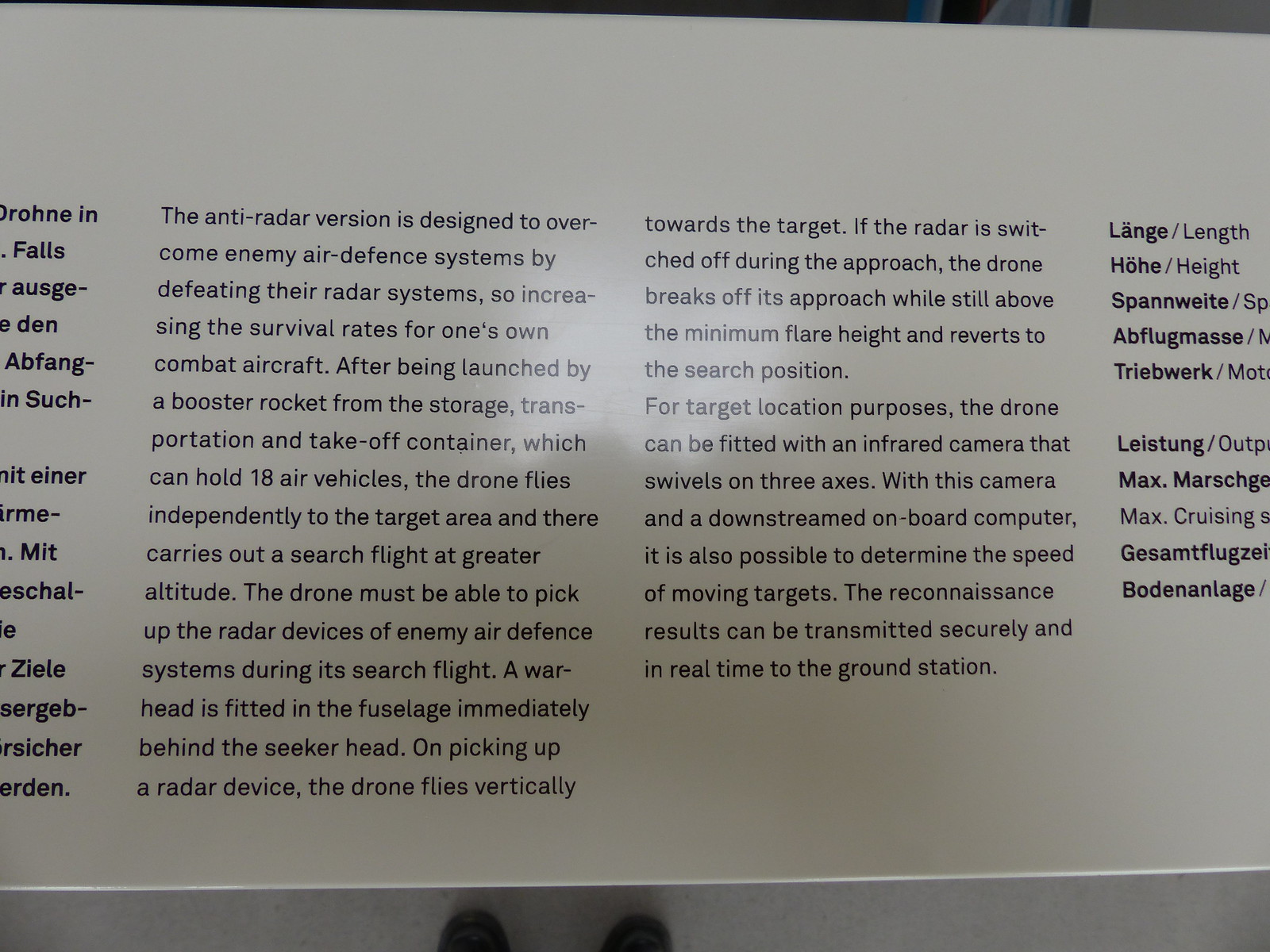This exhibit sign, displayed on a white background with black text, provides a detailed description of an anti-radar drone system designed to enhance the survivability of friendly combat aircraft by defeating enemy radar systems. The sign is divided into two main columns, with some initial words in another, unidentifiable language partially cut off at the extreme left. The English portion of the first column describes how the anti-radar drone is launched from a storage, transportation, and take-off container that can hold 18 air vehicles. Once launched by a booster rocket, the drone independently flies to the target area, performing a search flight at a higher altitude to locate enemy radar devices. The drone, equipped with a warhead behind its seeker head, ascends vertically towards the target upon identifying radar signals. The subsequent text in the second column details that if the radar is switched off during its approach, the drone reverts to its search position to resume scanning. For precise target acquisition, the drone can be fitted with a three-axis swiveling infrared camera and an onboard computer to detect and measure the speed of moving targets. Reconnaissance data is transmitted securely in real time to the ground station. The right side of the screen also features additional truncated text in dual languages, likely providing further context and confirming the bilingual nature of the information provided.